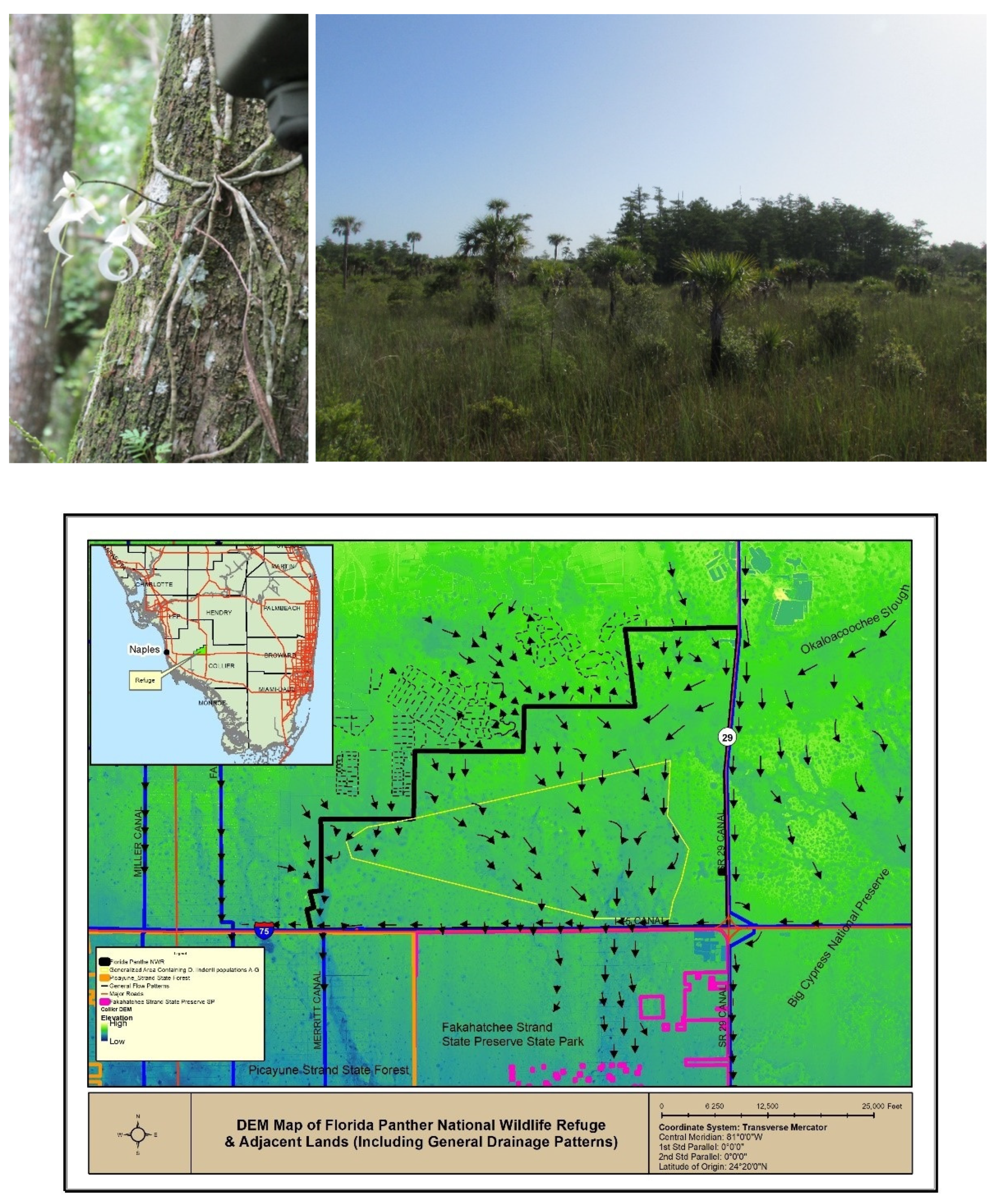### Detailed Descriptive Caption:

The image collage consists of three separate visual elements. At the top are two photographs placed side by side. The photograph on the left showcases a ghost orchid (Dendrophylax lindenii) clinging to the gray bark of a tree trunk. The orchid's intricate gray roots spread across the bark, collecting nutrients and condensation from the humid air. The orchid features two stunningly white flowers, each with a star-like shape and a distinctively long petal forming a throat. To the right, the second photograph captures a serene landscape in the wild, characterized by tall grasses interspersed with small shrubs and scattered scrubs. A grove of trees stands prominently against a clear blue sky, depicting the lush and untamed beauty of this natural habitat.

Below these photographs is a detailed 2D map of a specific section of Florida. In the top left corner of the map, an inset provides an aerial view of the southern half of Florida, with an indication of the location slightly inland from the west coast. The main portion of the map highlights the Panther National Wildlife Refuge, illustrated in green. Various arrows on the map denote regions where the endangered Florida Panther can be found, emphasizing the refuge's significance as a conservation area for this majestic species.